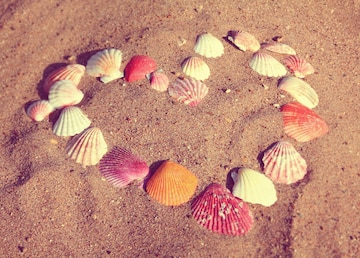Against the backdrop of a sunlit, tan-colored beach, this professionally-taken photograph showcases an artfully arranged heart made up of around 20 seashells in various shades, including white, off-white, yellow, pink, red, orange, and gold. Each shell, mostly clam-like in shape and size yet varying slightly, forms part of an intricately detailed motif. Displaying a counterclockwise rotation of about 20 degrees, the heart is composed of a mixture of solid-colored and patterned shells, some featuring spots or stripes. Scattered pebbles and debris dot the well-lit sand around the heart, adding texture to the scene. This captivating image beautifully captures the playful yet meticulous spirit of beach art, making it an ideal visual for a professional blog, magazine, or website article about seaside activities.